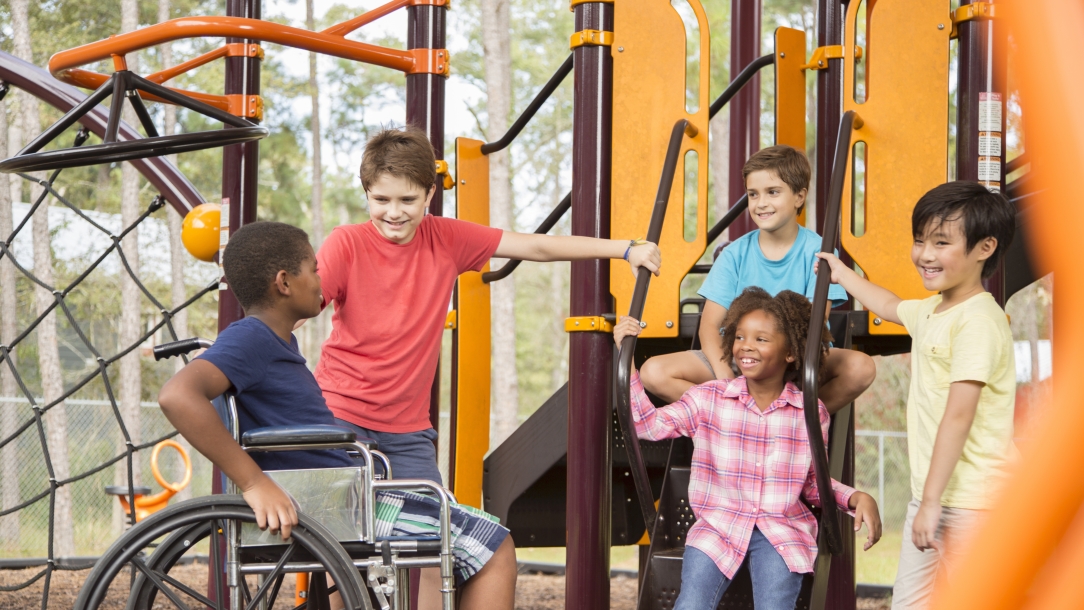This vibrant color photo captures five children of diverse backgrounds joyfully playing on an orange and brown playground structure. Prominently, a smiling black boy sits in a wheelchair, wearing a navy t-shirt and black, turquoise, and white striped board shorts. A white boy in a red t-shirt stands behind him, beaming, while two other white boys, one in a yellow shirt and khakis, and another in a blue shirt, play nearby. The fifth child, a black girl in a pink plaid shirt and blue jeans, is also visible. The playground features brown pillars, a slide, and a black spider-web-like climbing net. In the background, lush green trees, light foliage, and a metal chain-link fence are visible, as well as a rocking horse toy. The scene is filled with joy as all the children interact, highlighting the inclusive and cheerful atmosphere perfect for a magazine cover.